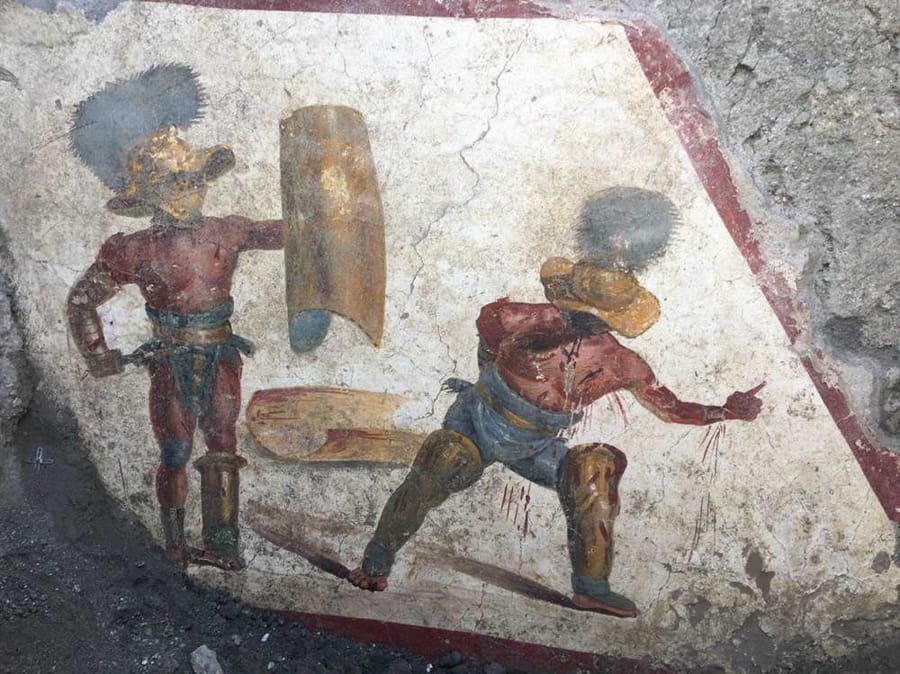The image showcases a detailed, full-color photograph of an ancient Roman painting, depicted on a weathered white stone surface tinged with shades of gray and black as if covering from dirt. The square artwork, which appears to be aging and slightly worn, portrays two Roman gladiators engaged in battle. In the upper right corner, gray rock is visible, while the lower left corner shows black mud-like residue. 

In the center of the painting, the gladiator on the left stands tall, poised with one hand on his hip and a curved golden shield in the other. This figure is attired in a red uniform complemented by a blue cloth wrapped around the waist and legs, and golden boots. The helmet is adorned with large gray feathers, adding a majestic appearance. He also holds a dagger in his right hand.

In stark contrast, the gladiator on the right is crouched and lunging forward, his right arm behind his back while his left arm, now severed, lies bleeding. His shield rests discarded on the ground. Similar to his opponent, he is dressed in a blue cloth around the waist, golden leg armor, and a round golden helmet with fuzzy gray ornaments. The backdrop reveals a stone surface with visible cracks, enhancing the painting's antique and rugged nature.